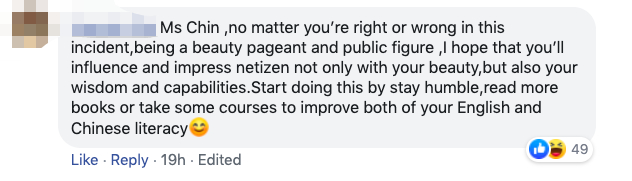This image features a screenshot of a Facebook comment. Both the profile image and the user's name are pixelated for privacy. The comment appears in a light gray text bubble with black text and reads:

"Ms. Chin, no matter if you're right or wrong in this incident, being a beauty pageant and public figure, I hope that you'll influence and impress netizens not only with your beauty but also your wisdom and capabilities. Start doing this by staying humble, reading more books, or taking some courses to improve both your English and Chinese literacy 😊."

The comment has received a total of 49 reactions, including thumbs up and laughing emojis. Below the comment, there are interactive links, 'Like' and 'Reply,' and it notes that the comment was posted 19 hours ago and has been edited.